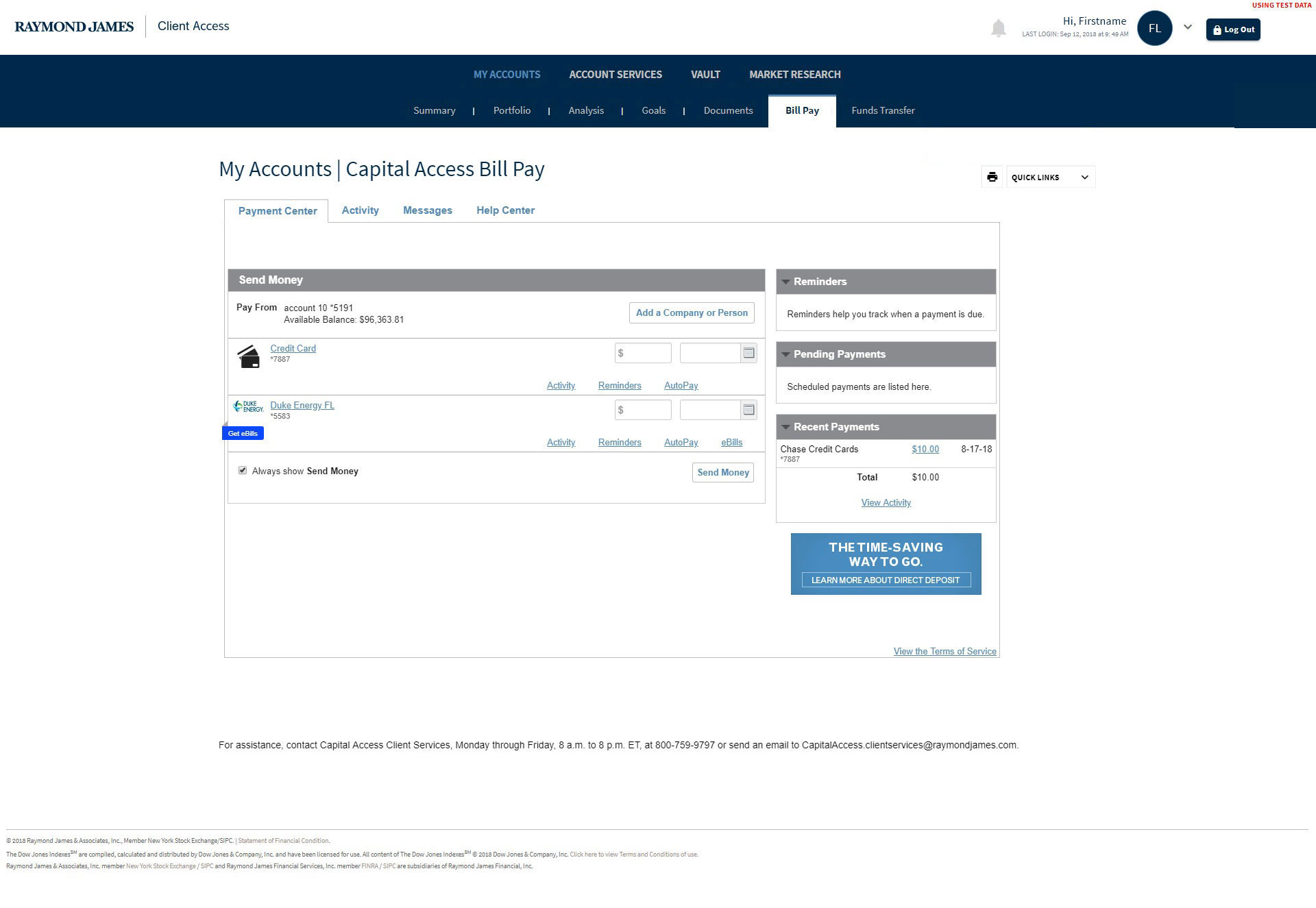The screen capture from the Raymond James webpage features a detailed user interface for the "Client Access" section, prominently displayed in the upper-left corner. In the upper-right corner, there is a login field for users. The primary focus of the capture is the "My Accounts" section, specifically highlighting the "Capital Access Bill Pay" functionality.

In the main field, four tabs are visible, with the "Payment Center" tab currently selected. The other tabs include "Activity," "Messages," and "Help Center." Under the "Payment Center" tab, users have various options for sending money. There is an option to add a company or person, which is adjacent to the partial entry for a credit card number, alongside fields for the amount and date of the transaction.

Below this, we can see a bill entry for "Duke Energy FL," potentially indicating a utility payment. Similar fields are present here, including those for the bill number and date. To the far right, there are sections for reminders, pending payments, and recent payments.

The upper ribbon of the interface indicates that users are in the "Bill Pay" section, as evidenced by the highlighted "Bill Pay" option among other navigation choices such as "Summary," "Portfolio," "Analysis," "Documents," and "Fund Transfer." The overall presentation suggests a comprehensive money management tool designed for efficient bill payments and financial oversight.